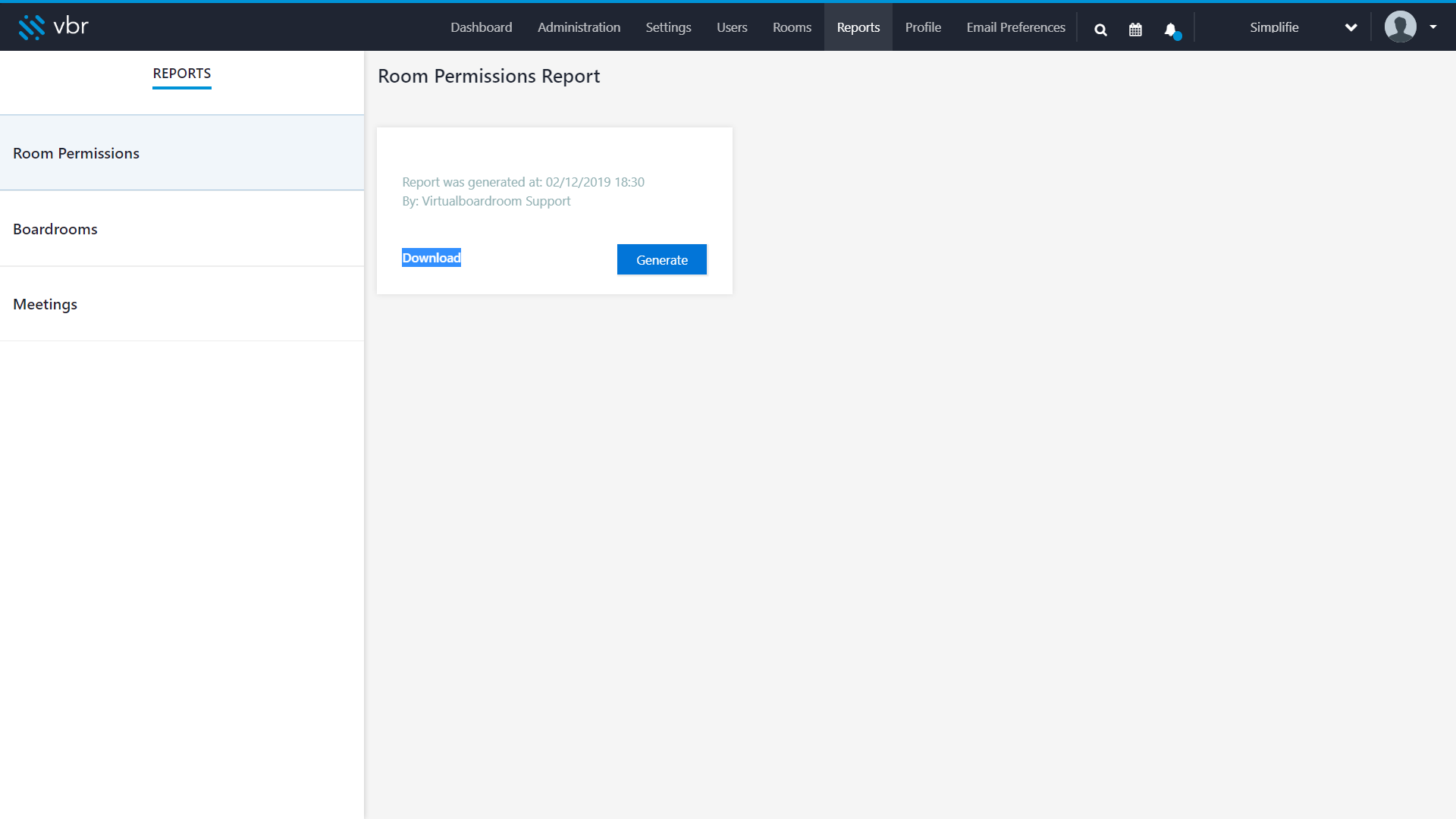The image is a screenshot from a desktop or laptop, characterized by its widescreen, rectangular dimensions. The interface primarily features a light background, with a column on the left side occupying about a fifth to a quarter of the image. This column has a white background. The rest of the screen to the right displays a light grey background.

At the top of the screen, there's a nearly black, dark blue header. On the left side of this header, there is a blue logo composed of simple blue lines forming a square, accompanied by the lowercase letters "vbr" in white—presumably indicating the company's name.

The header contains clickable links for various sections: Dashboard, Administration, Settings, Users, Rooms, Reports, Profile, and Email Preferences. The "Reports" tab is currently selected, highlighted to distinguish it from the others.

Below the header, the text "Room Permissions Report" is displayed. A white prompt beneath this text states, "Report was generated on 2/12/2019 at 18:30 by Virtual Boardroom Support." Below the prompt, there are two blue buttons labeled "Download" and "Generate."